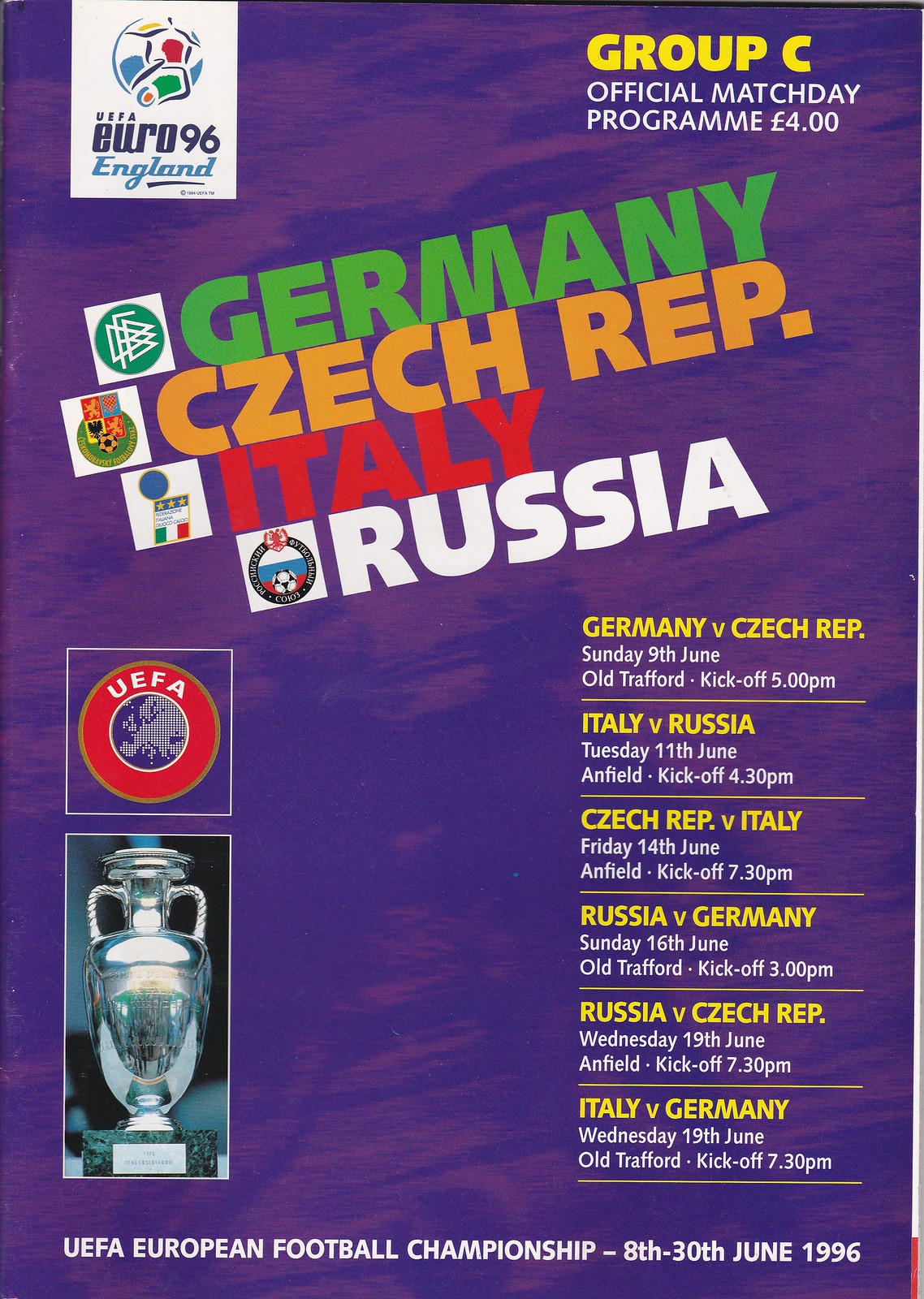The image is a vibrant advertisement or flyer, potentially a match day program for the UEFA Euro 96 tournament, Group C. It features a purple, somewhat grungy background with light purple splotches scattered across. Prominent text in the upper right-hand corner states, "Group C Official Match Day Program, $4." The upper left-hand corner displays the UEFA Euro 96 England logo.

Centrally, bold colored texts list the participating teams: "Germany" in green, "Czech Republic" in yellow-orange, "Italy" in red, and "Russia" in white, each accompanied by their respective logos, flags, and emblems. Below the team names, on the left, there's a UEFA logo in red, white, and blue, with a bordered picture of a silver trophy beneath it.

On the right side, yellow and white text outlines the match-ups: Germany vs. Czech Republic, Italy vs. Russia, Czech Republic vs. Italy, Russia vs. Germany, Russia vs. Czech Republic, and Italy vs. Germany. Each match listing includes the date, location, and kickoff time details. At the very bottom, white text reads, "UEFA European Football Championship, 8th through 30th June 1996."